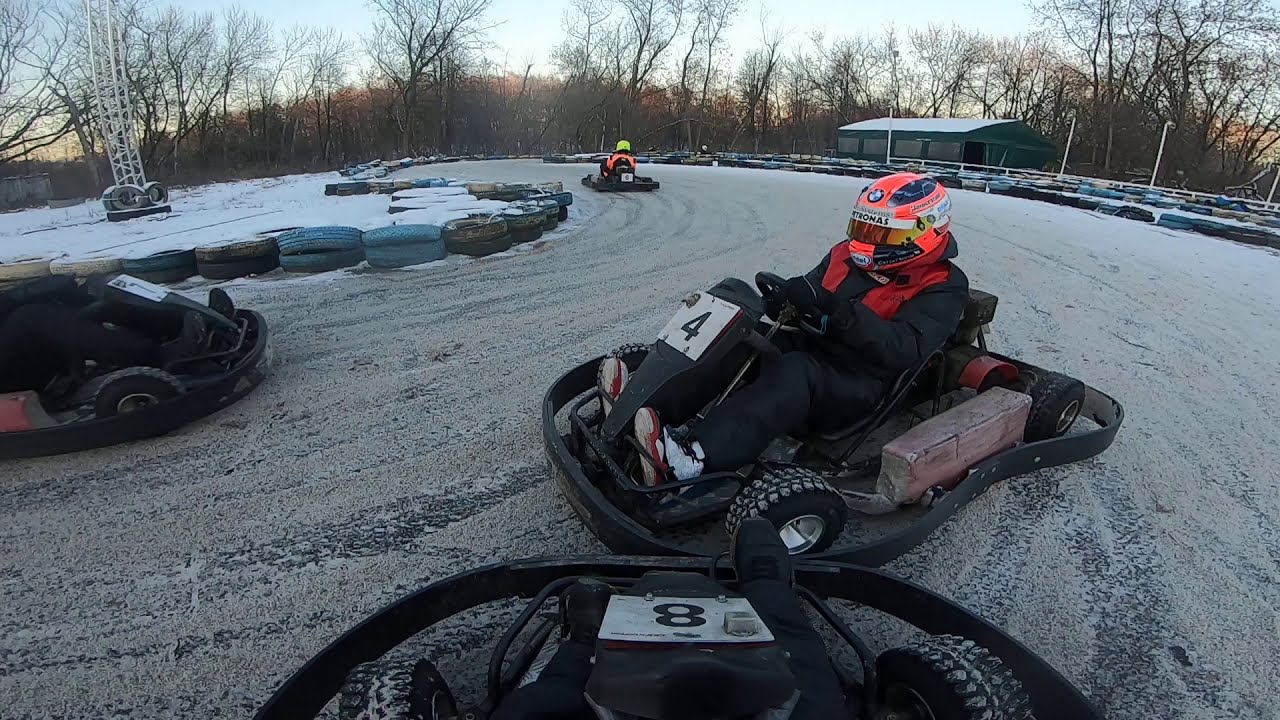The image captures an outdoor go-kart track teeming with activity, possibly involving kids or young adults racing. At the center of attention is a black go-kart numbered 4, driven by an individual wearing an orange and black-striped helmet, matched by a similarly colored shirt. There are other racers visible; one in the distance seems to sport similar attire, and another, partially visible go-kart appears at the far right of the frame, identifiable by its back wheels and similar coloration. 

The track, composed of mixed white and black gravel, is encircled by tires outlining its perimeter. A distinctive round feature in the middle, possibly covered with snow and encircled with baffles, stands out prominently. The backdrop reveals a green outbuilding, bare trees suggestive of winter, and a potential mountainous area cloaked behind the tree line. 

The scene unfolds under a clear daytime sky with minimal clouds, and all participants are outfitted with helmets and winter attire, including jackets and gloves, indicative of the chilly season. The go-karts, evidently rentable and numbered, hint at a well-maintained and sizeable track designed for thrilling rides, with turns and twists stretching off into the distance.